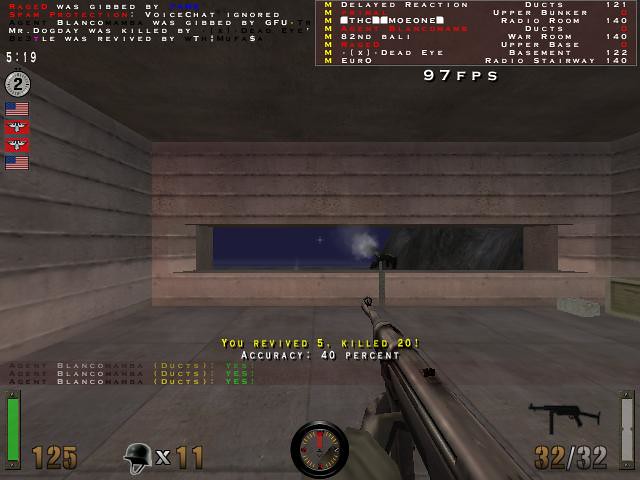The image is a detailed screenshot from the game "Return to Castle Wolfenstein." It shows a first-person view of a soldier inside a large brick bunker room with a long, rectangular shooting window at the back. The scene features a dark blue sky and a mountain visible through the window. The soldier's left hand is clasping the barrel of an MP44 rifle, which is pointed toward the window. 

The image showcases the game's user interface. In the top right corner, there's a box displaying various names and words, with "97 FPS" (frames per second) noted below. At the bottom right, there's a gun icon showing the ammunition count as "32/32." The bottom left displays a vertically positioned green status bar marked with "125" next to it, and a helmet icon indicating "11." Centered on the screen are the statistics "You revived: 5, Killed: 20, Accuracy: 40%," indicating the player's performance for the finished game. The overall color scheme includes yellows, reds, and whites, providing various UI elements.